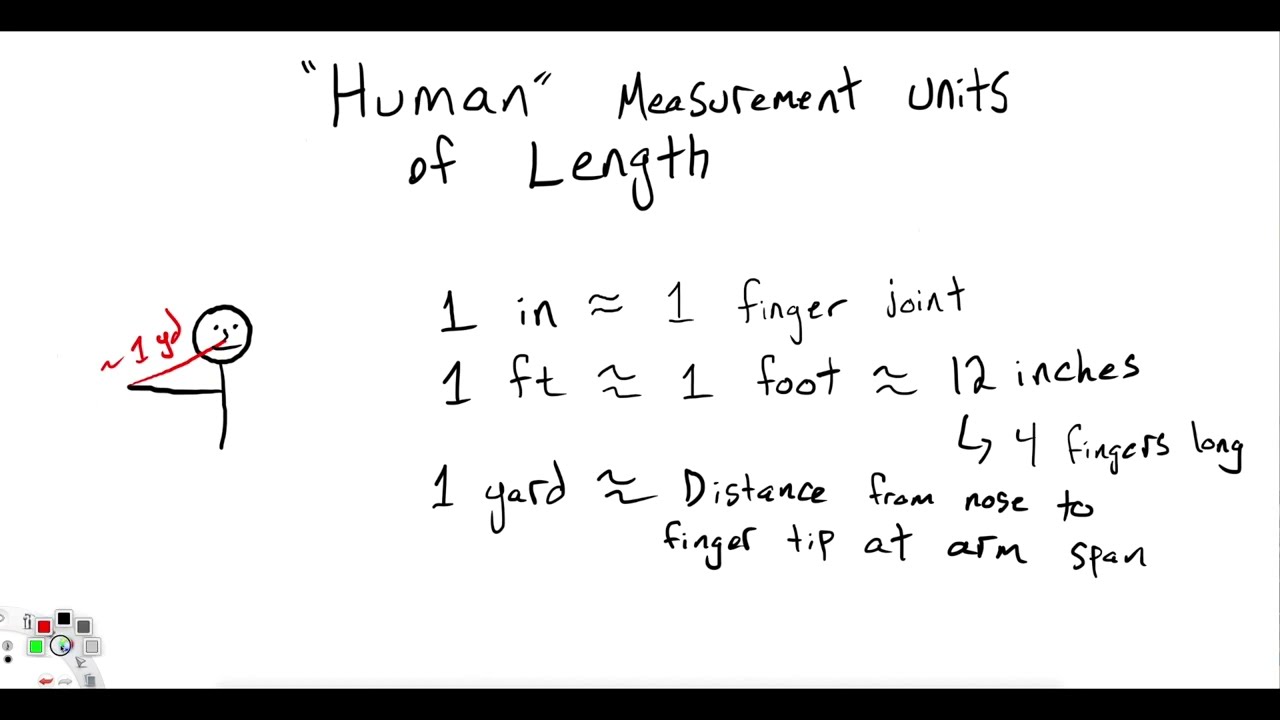The image depicts an educational whiteboard designed to explain human measurement units of length. At the top of the whiteboard, set against a black banner, it reads in quotation marks: "human measurement units" followed by "of length." The board features a central stick figure with a single outstretched arm to the right. To the left of the stick figure is a mathematical symbol marked "1 YD" underlined in red, with a red line connecting the figure's arm to its nose, indicating the span. Below the main title, the whiteboard details: "1 inch equals one finger joint," "1 foot equals one foot or 12 inches," and "one yard equals the distance from nose to fingertip or arm span." Additionally, there is an annotation pointing to "four fingers long" with an arrow directed downward and to the right. In the bottom left corner, there is a colorful logo or set of icons, although their specifics are unclear.